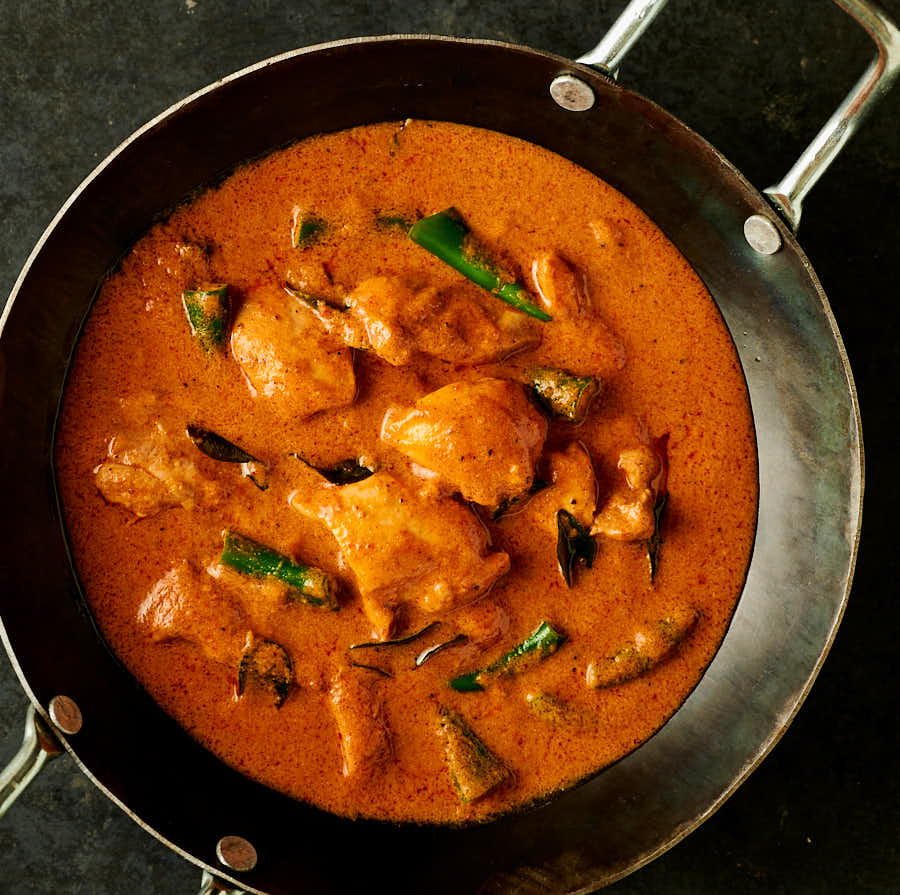A bird's-eye view photograph captures a mouthwatering scene in a well-used black iron skillet with metal handles, placed on a dark countertop. The amber-orange curry, possibly butter chicken, bubbles gently, releasing tantalizing aromas. Chunks of chicken are prominently visible, nestled in the rich, flavorful sauce. Adding complexity, the dish includes potential mussels, identifiable by their black shells. Bright green whole larger chilies and possibly some beans or asparagus slices are scattered throughout, contributing both color and a hint of spiciness. The greenery forms a ring along the periphery, with a few pieces mingling amidst the central chicken chunks, creating a visually appealing and inviting meal.